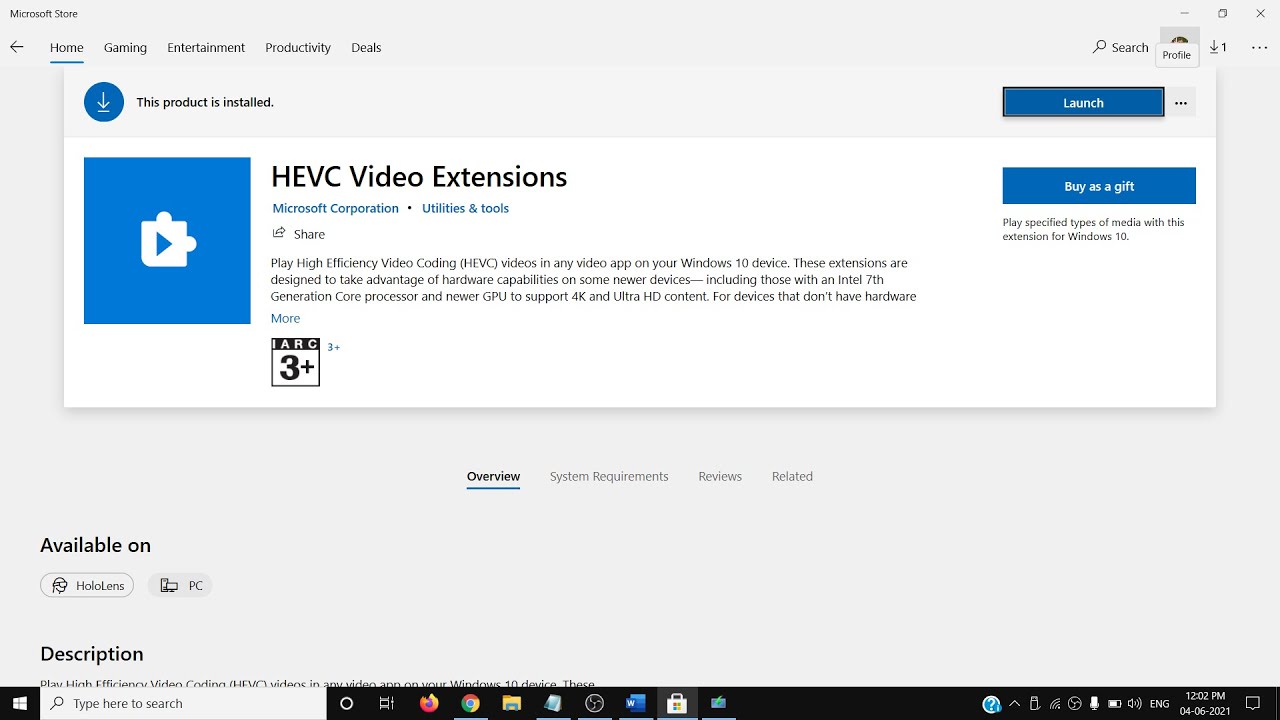The image appears to be a screenshot from a Microsoft Windows laptop with the Microsoft Store application open. 

At the bottom of the screen, the Windows taskbar is visible, featuring various icons and elements. From left to right, the taskbar includes the Windows Start menu icon labeled "Type here to search," followed by icons for Power, Notifications, Firefox, Google Chrome, File Explorer, Notepad, Microsoft Word, and potentially Excel, represented by a green icon. There is a gap, after which the taskbar displays system tray icons including the time, battery status, and language settings, showing "English," the time "12:02 PM," and the date "4-6-2021," indicating that the screenshot is from an older date.

The main focus of the screen is the Microsoft Store app, specifically under the "Home" section. The featured product is "HEVC Video Extensions" by Microsoft Corporation. The description states that these extensions enable playing High Efficiency Video Coding (HEVC) videos in any Windows 10 video app. It is noted to be suitable for ages 3 and up and available on HoloLens and PC.

The product is shown as "Installed," with options to "Buy as gift" and "Launch." There is a search bar at the top. Below, the description further explains that these extensions are designed to leverage hardware capabilities of newer devices, particularly those with an Intel 7th generation core processor and newer GPUs, to support 4K and Ultra HD content. The description includes a mention that for devices lacking the necessary hardware, these benefits may not apply.

In the upper right-hand corner of the screen, the user profile icon is partially obscured by the word "Profile". Adjacent to it is a notification showing "Downloads (1)" and a series of three symbols typically used for settings and additional options.